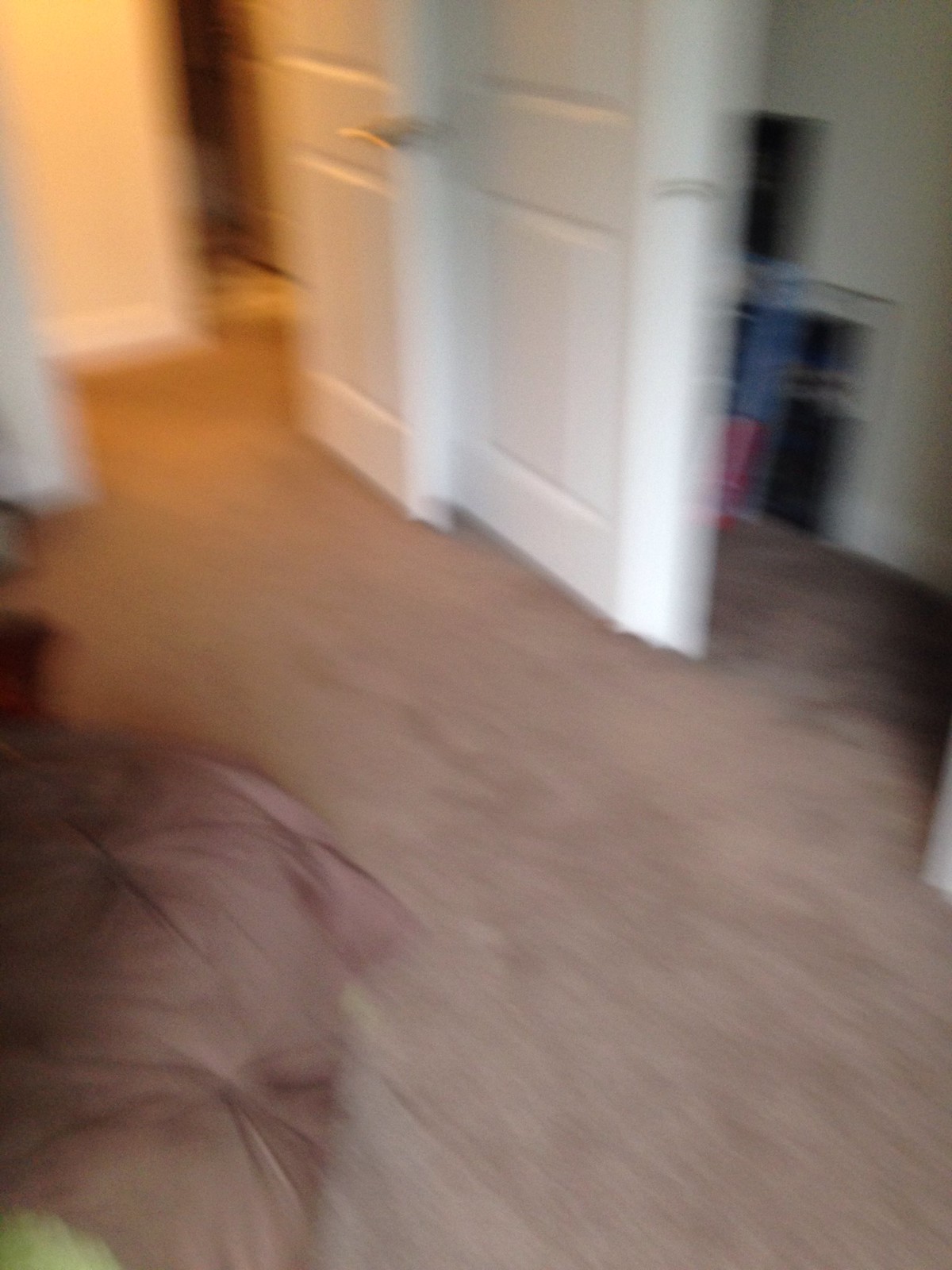This blurry photo, likely taken inside a house and possibly in a bedroom, captures a somewhat chaotic and unclear scene. The room features a light brown carpet, which extends into a brightly lit hallway. The hallway leads to another room with what appears to be linoleum flooring. Two white doors are present; one is a typical door while the other seems to be a closet door. The doorknobs are golden bars. Several objects are scattered on the floor: a patterned darker brown object, a bulky pink-like item (possibly a blanket or comforter), and a speck of light green in the bottom left corner. Additionally, there are a few more items visible: a blue item, a pink item, and two black ones. The walls within the room are a cream white color, adding some brightness despite the low-quality image that was likely taken hastily. At the top center of the photo, the open doors lead to a hallway, enhancing the sense of depth in the room.